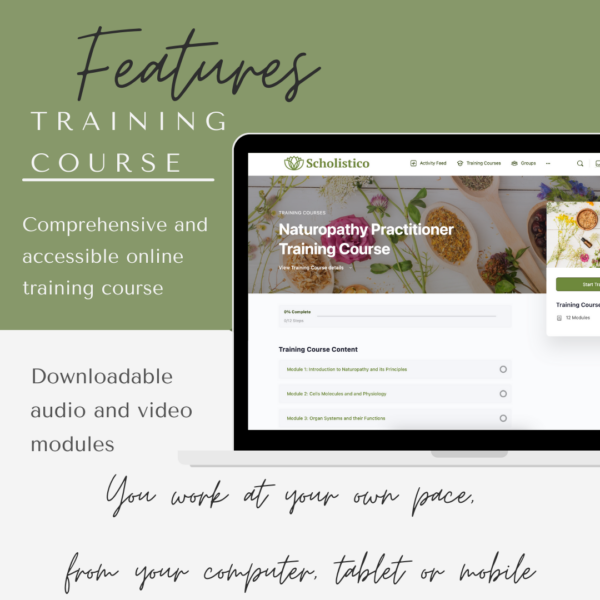The top portion of the image features an olive green background with the word "Features" elegantly written in black cursive. Below this, "TRAINING COURSE" is displayed in uppercase white letters, underlined for emphasis, followed by the description "Comprehensive and accessible online training course." 

On the right side of the image, an outlined black frame resembles the exterior of an iPad or laptop screen. At the top of this frame, in green text, is the title "SCHOLISTICO." Below it, there are images depicting various spoons filled with different herbs, along with green plants and herbs placed on a counter surface. Above these images, the text reads "Naturopathy Practitioner Training Course."

To the left side of the image, there is an indication for "Download or downloadable audio and video modules." Below this, in cursive writing, are the words "You work at your own pace," and at the very bottom in black cursive, it states, "from your computer, tablet, or mobile."